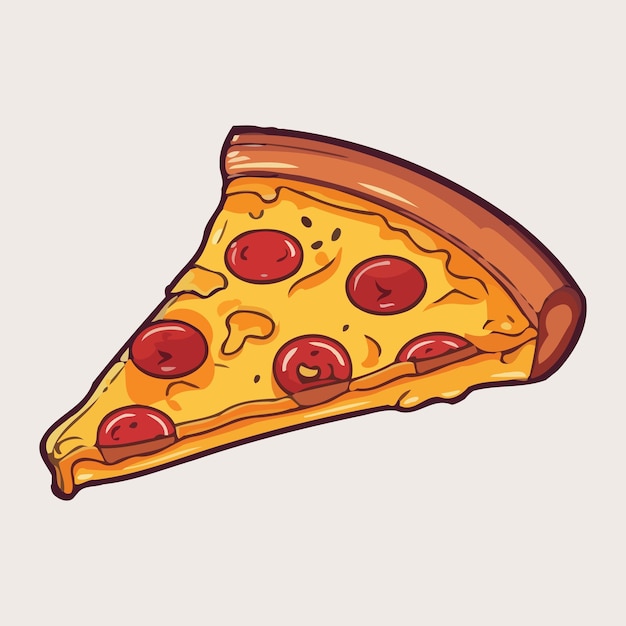This is a detailed computer-generated illustration of a slice of pepperoni pizza rendered in a cartoonish style. The focal point of this artwork is the thick-crusted slice, prominently featuring six evenly spread red pepperoni slices. The cheese, depicted in various shades of yellow and orange, appears to be melting generously down the sides and front of the pizza. The crust, showcased at the back of the slice, is illustrated in a beige and brown hue and interestingly contains a noticeable hole. Accentuating the slice, the artist has used a dark, bold outline, enhancing the defined look of the pizza and adding depth to the graphic. Moreover, inside the pizza slice, black lines meticulously differentiate various elements. The illustration also includes smaller black specks scattered across the pizza, resembling seeds or possibly seasoning like oregano. The backdrop of this image is a light grayish-beige color that contrasts well with the vivid colors of the pizza, emphasizing its visual appeal.